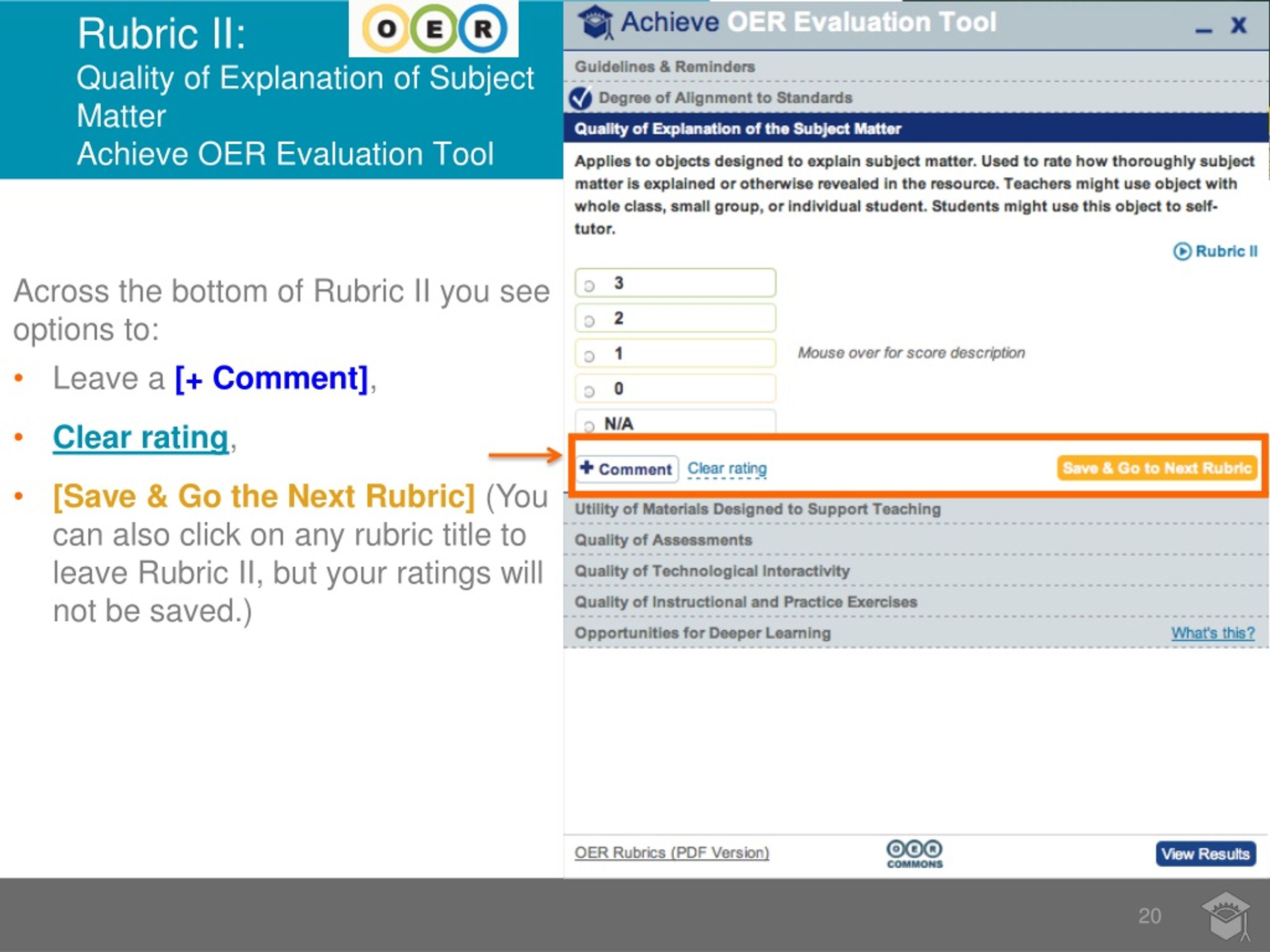The image features a screenshot set against a white background. In the upper left corner, there is a blue box labeled "Rubric 2: Quality of Explanation of Subject Matter." To the top right of this box is the OER logo, followed by a gray box containing the word "Achieve" accompanied by a blue graduation hat icon.

The screenshot elaborates on the OER (Open Educational Resources) evaluation tool, providing guidelines and reminders. It focuses on the "Degree of Alignment to Standards" and the "Quality of Explanation of the Subject Matter." The rubric is intended for evaluating resources designed to explain subject matter and is used to rate how thoroughly the subject matter is explained or revealed in the resource.

Teachers might use this evaluation tool with a whole class, small groups, or individual students. Similarly, students might use the object for self-tutoring. Across the bottom of Rubric 2, there are options available to leave a comment.